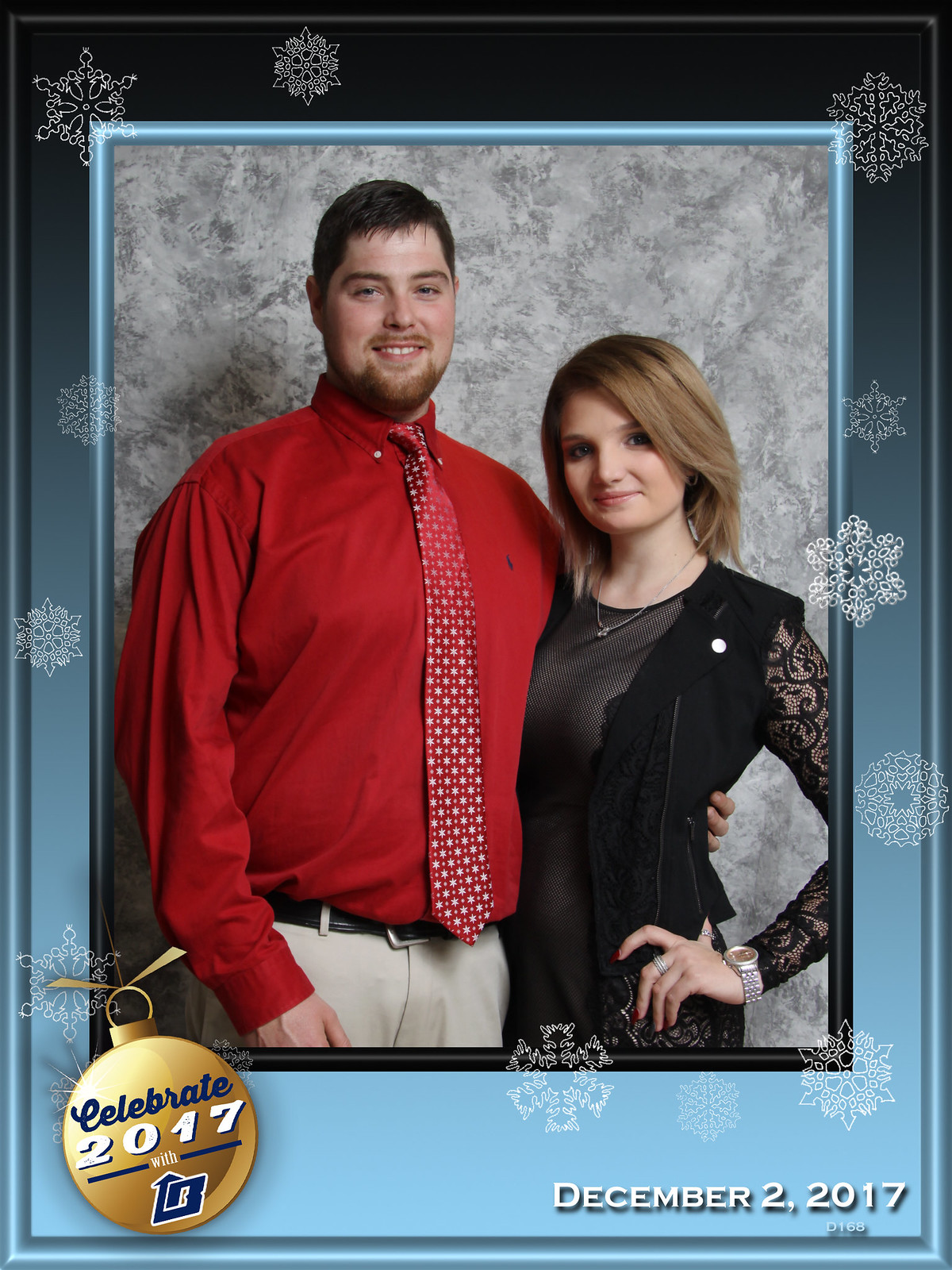The image features a man and a woman posing against a wintery-themed backdrop, suggesting a holiday or Christmas celebration, as marked by the snowflakes adorning the black-to-blue gradient border. A golden ornament is placed in the bottom left corner, inscribed with "Celebrate 2017" alongside a logo featuring a 'B' with an upward arrow. The bottom right corner displays the date "December 2nd, 2017." The man is dressed in a red shirt complemented by a red polka dot tie and gray slacks, accessorized with a black belt. He has dark hair, a mustache, and a beard. The woman dons an elegant black dress with lace sleeves and wears accessories including a necklace, watch, and ring on her second finger. She has brown hair. The overall scene evokes a festive, wintery atmosphere.